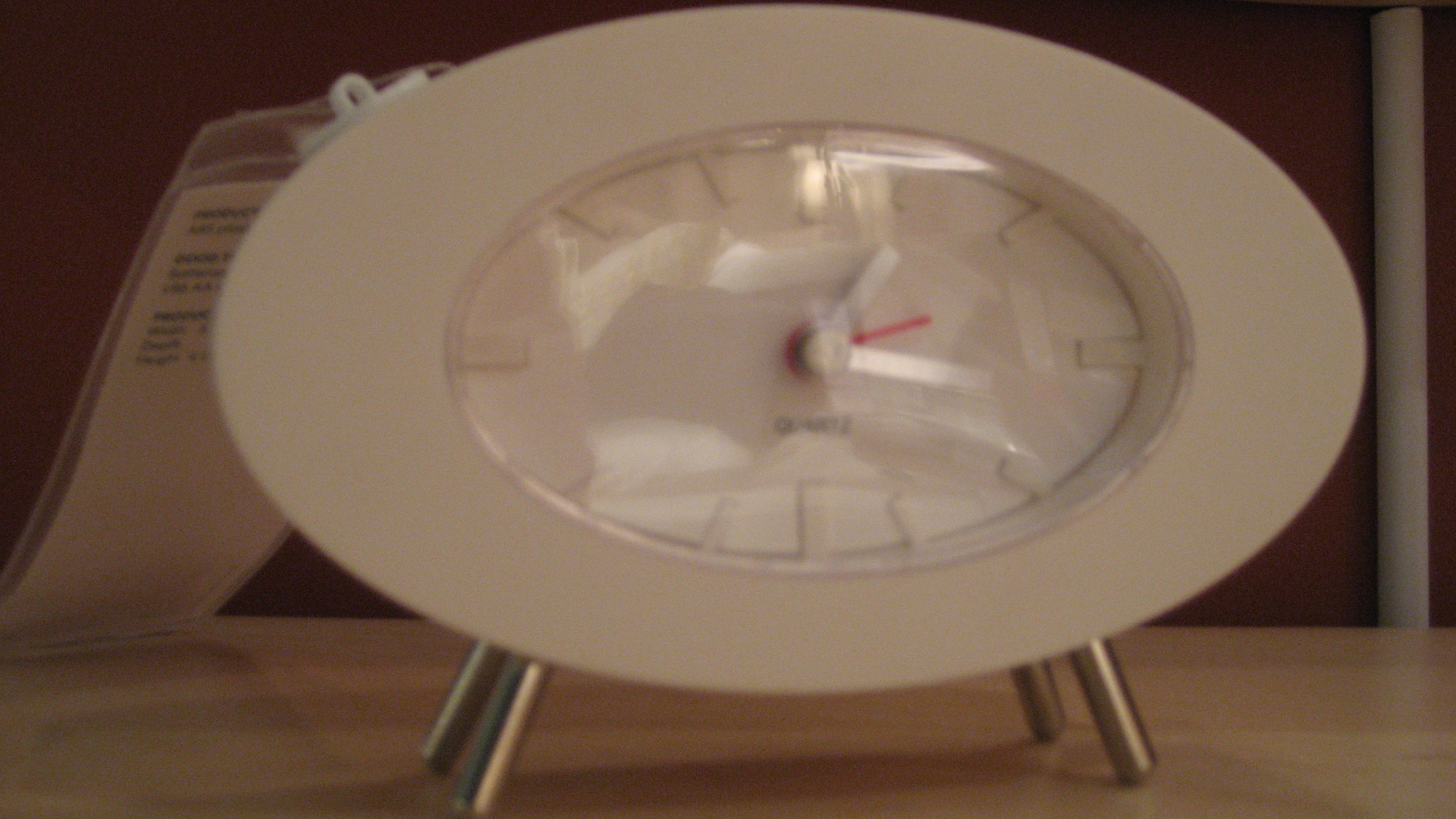In the image, an analog clock with an oval, eggshell-white body sits prominently on a walnut-colored tabletop, supported by four small silver legs. The clock features a distinctive, thick border and has a reflective glass face with a glare caused by the ceiling light. Behind the clock, the background is a rich, dark brown wall with a gray lining. The clock's hands are partly obscured but are identifiable as a white minute and hour hand, complemented by a bright red second hand. Instead of numerals, the clock face displays white lines indicating the hours. A white round pipe is positioned behind the table, leaning against the wall. Attached to the clock are three pieces of paper resembling a price tag, although the text on them is unreadable. This unusual, space-age looking desktop clock brings a touch of modernity to a classic style.